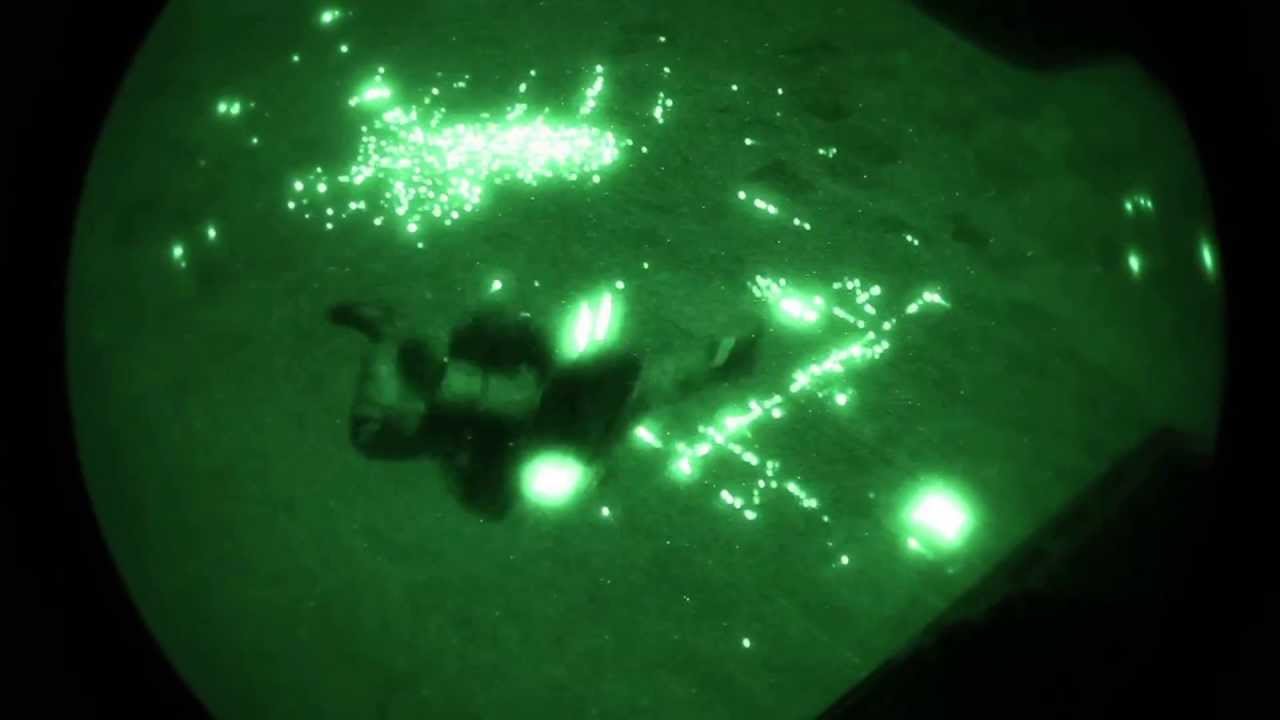In this rectangular, six-inch-wide by three-inch-tall image, captured through what appears to be a night vision lens, the focal point is an expansive green area shaped like a light bulb lying on its side, set against a stark black background. The upper left quadrant of this green 'light bulb' area is densely populated with clusters of bright, white lights that resemble a swarm of fireflies or perhaps city lights viewed from above at night. Beneath this cluster, a dark, blurred figure emerges, giving the impression of a person in freefall—potentially a skydiver—arms and legs splayed outwards. To the bottom right of the figure, a series of bright lights form a linear pattern reminiscent of runway lights, enhancing the aerial perspective while adding additional intrigue and movement to the scene. The image, though blurry and indistinct, evokes the feeling of looking at a still frame from a night-time skydive video, dominated by contrasting green and black hues, and speckled with splotches of light and distorted reflections.